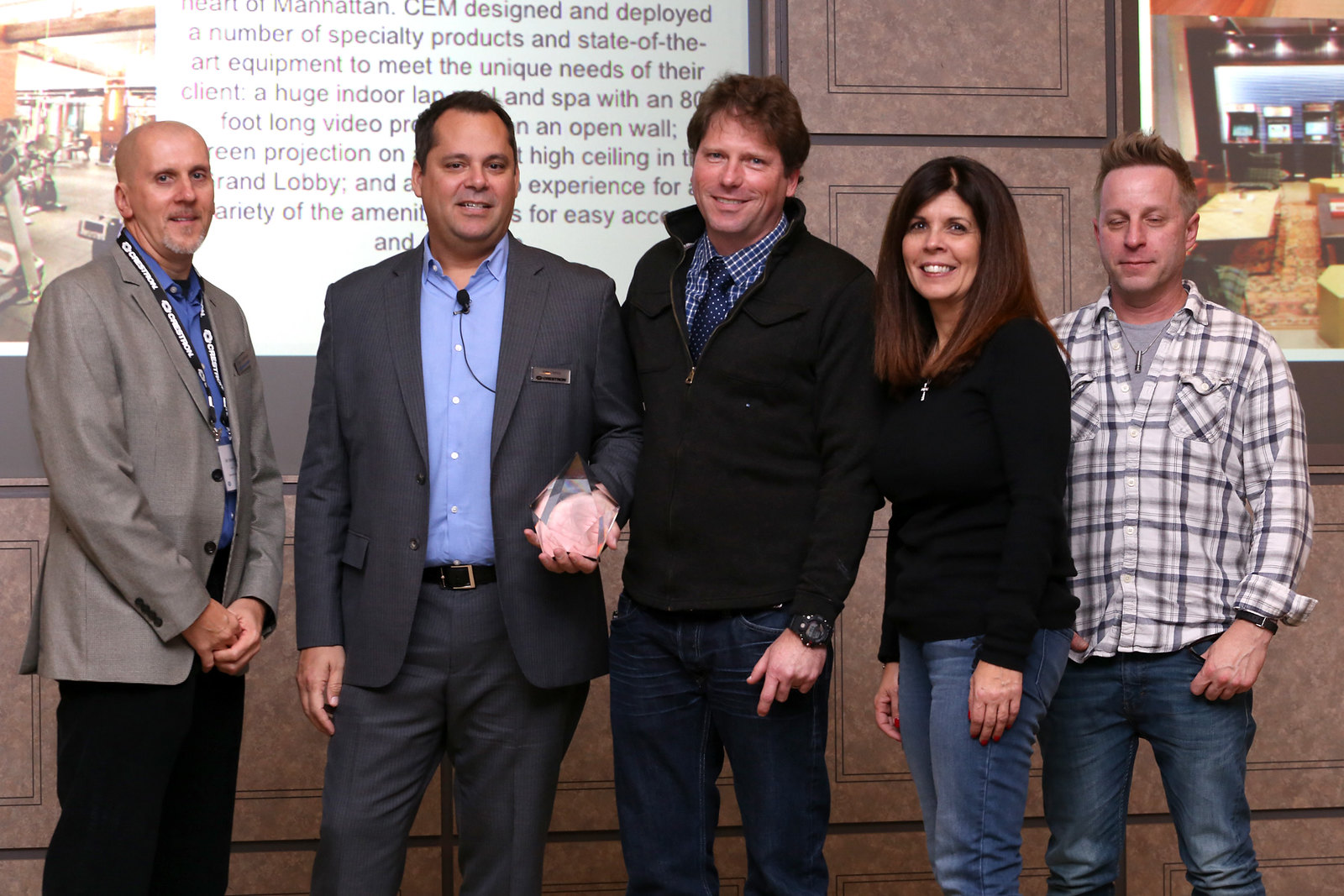In this image, a group of five people, consisting of four men and one woman, are posing together in front of a brown and black tiled wall adorned with various posters and a white square sign with black text that partially reads: "Heart of Manhattan, CEM, designed and deployed a number of specialty products and state-of-the-art equipment to meet the unique needs of their client." The individual on the far left is a bald gentleman wearing a gray suit and a blue lanyard, holding up a pink and gray piece of paper. Next to him is another man in a blue shirt, black suit, and a gold-buckled belt, holding a microphone and with a name badge around his neck. In the center stands a man in a black blazer over a spotted blue shirt and blue pants, holding hands with the man next to him, who is wearing a checkered shirt, tie, and watch. To the right of him is a woman with long dark brown hair, dressed in a black shirt and jeans. Lastly, the man on the farthest right is wearing a plaid shirt over a gray shirt and blue jeans, with his eyes closed. The group is standing against a backdrop with large photographs and posters that are partially obscured by their presence.